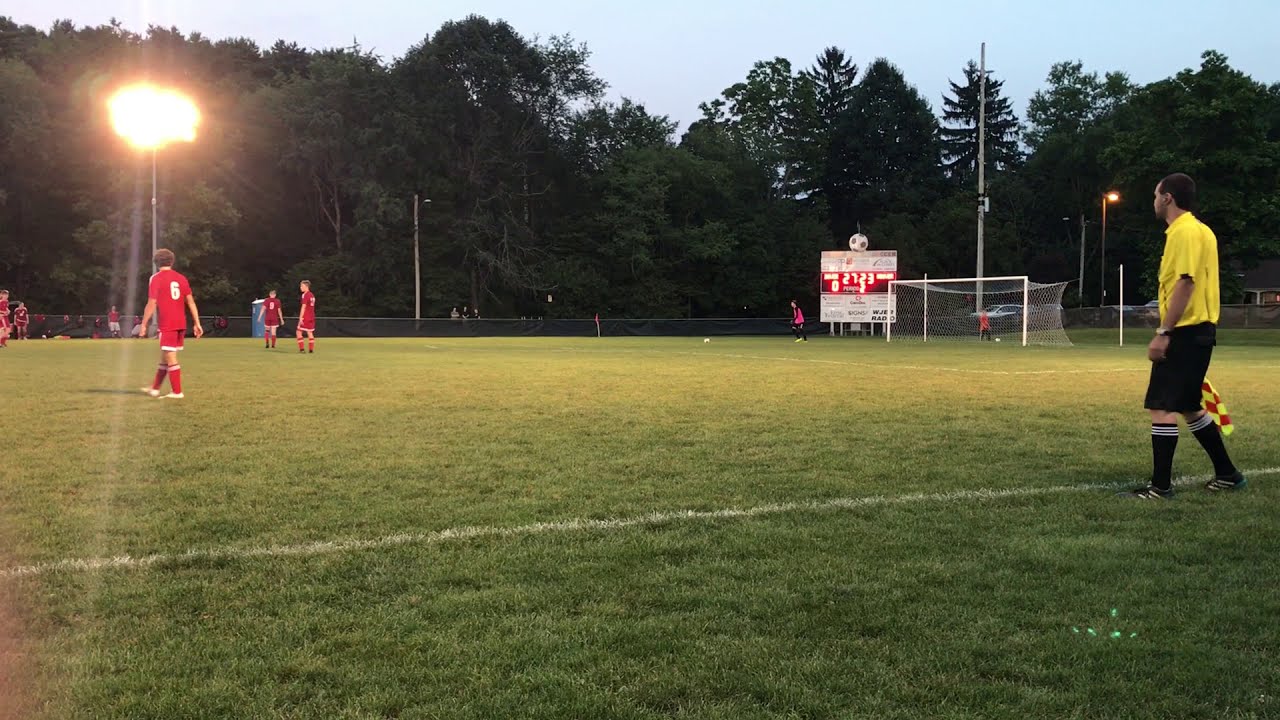In this detailed image of a soccer game, the scene is set during twilight, either at dawn or dusk. The soft light from the setting or rising sun casts a glow over the field, where the match is taking place under the illumination of large stadium lights. Dominating the foreground is a referee, easily identified by his bright neon yellow shirt, black shorts, knee-high black socks with white stripes, and black shoes accented with white. He holds a flag with alternating yellow and red squares, standing just outside the field lines on the right side of the image.

The background reveals a lush treeline encircling the field, with tall trees visible on the right side. Near the top right of the image, a soccer goal stands in front of an electronic scoreboard, which displays a score of 0 to 2 and a time reading between 27 and 23. Although finer details of the scoreboard are unclear, above it, a decorative imitation of a soccer ball is perched.

Gathered mainly on the left side of the image are the young players, clad in red jerseys, shorts, and high socks with white accents at the tops. One particular player, wearing the number 6 on his jersey, stands closest to the camera with his back visible. The remaining players, some standing and others seated, linger near the edge of the field, ready for their turn to engage in the match. The scene includes other background elements such as scattered vehicles, additional lights, and poles, contributing to the overall lively atmosphere of this youth soccer game set amidst a picturesque twilight.